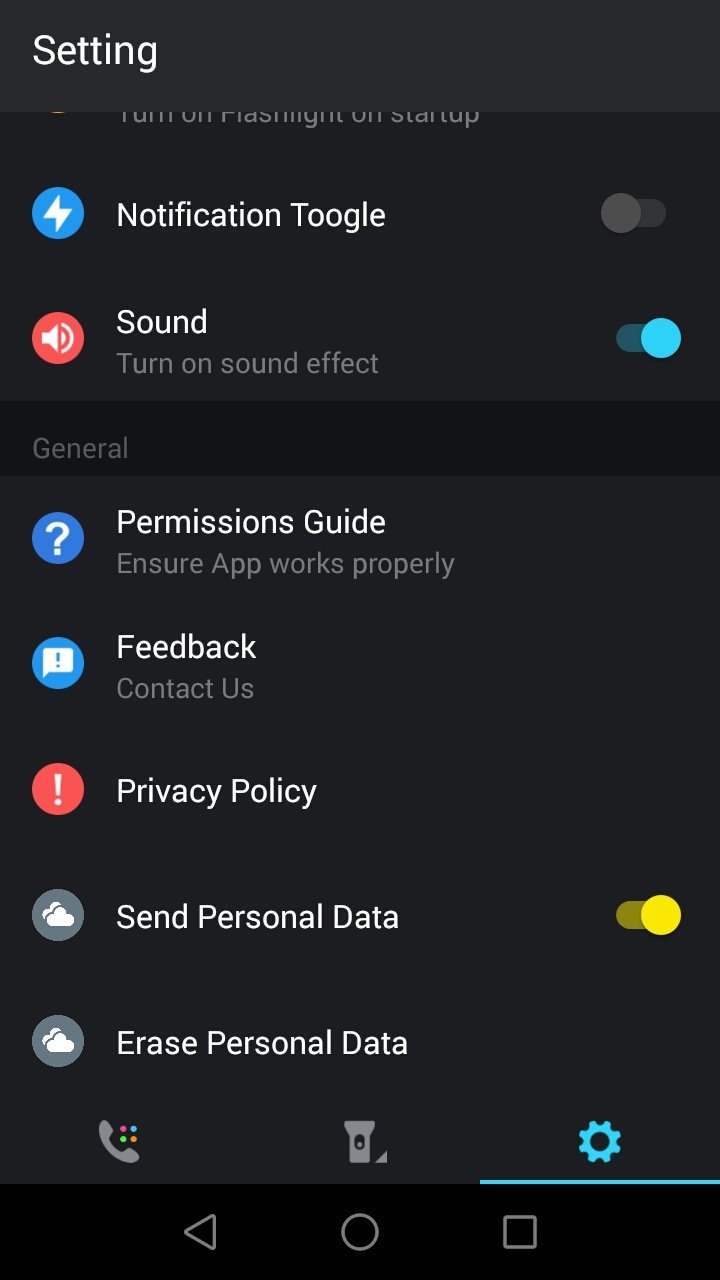The image showcases a variety of settings and toggles within an app interface, presumably under the "Tonset" settings section. Prominently featured is a blue circle associated with a notification toggle in an inactive state. Nearby is a red circle labeled "Sound," with an accompanying toggle for "Sound Effects." There is also a "General Permissions Guide" provided to ensure the app functions correctly.

Adjacent to these elements, another blue circle includes an icon resembling a speech bubble, accompanied by options for "Feedback" and "Contact Us." A red circle marked "Privacy Policy" is present, and a gray circle says "Erase Personal Data." Users can manage flashlight settings through a dedicated toggle.

The remainder of the interface includes several gear icons, suggesting settings or configuration menus. Additional navigational elements include a left-pointing triangle, variously colored circles, a square, and a black horizontal bar at the bottom, which likely serves as a separator or footer in the design.